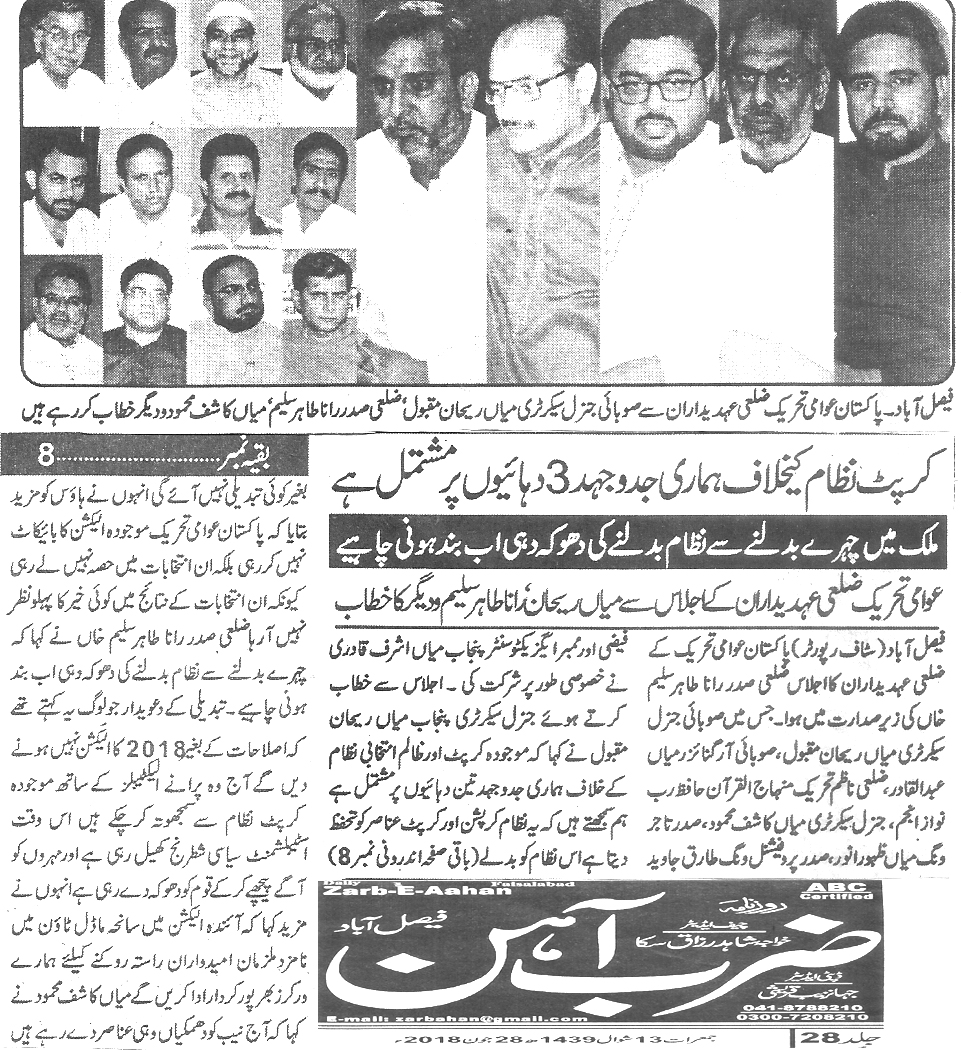The image is a black and white page from an Arabic newspaper dated 2018. Along the top portion of the page is a series of portraits of men, arranged in a grid. On the left side, there are 12 small, almost square, portraits organized into three rows and four columns. These photographs feature men, many of whom have beards or mustaches and dark hair, looking in various directions. To the right of this grid are five larger, vertically rectangular portraits that show not only the faces but also the torsos of the men. 

Below these images is a significant amount of Arabic text. On the left side, the text includes a paragraph clearly mentioning the year 2018. The right section of the text consists of two paragraphs highlighted by black backgrounds with white text, possibly indicating subheadings or important sections. At the very bottom of the page is a small advertisement with the words "Zabi Han, ABC certified" accompanied by large Arabic characters, an email address, a phone number, and a sequence of numbers, including a date reference "2018, 28, 14, 39, 13." The bottom of the page indicates that it is page 28.